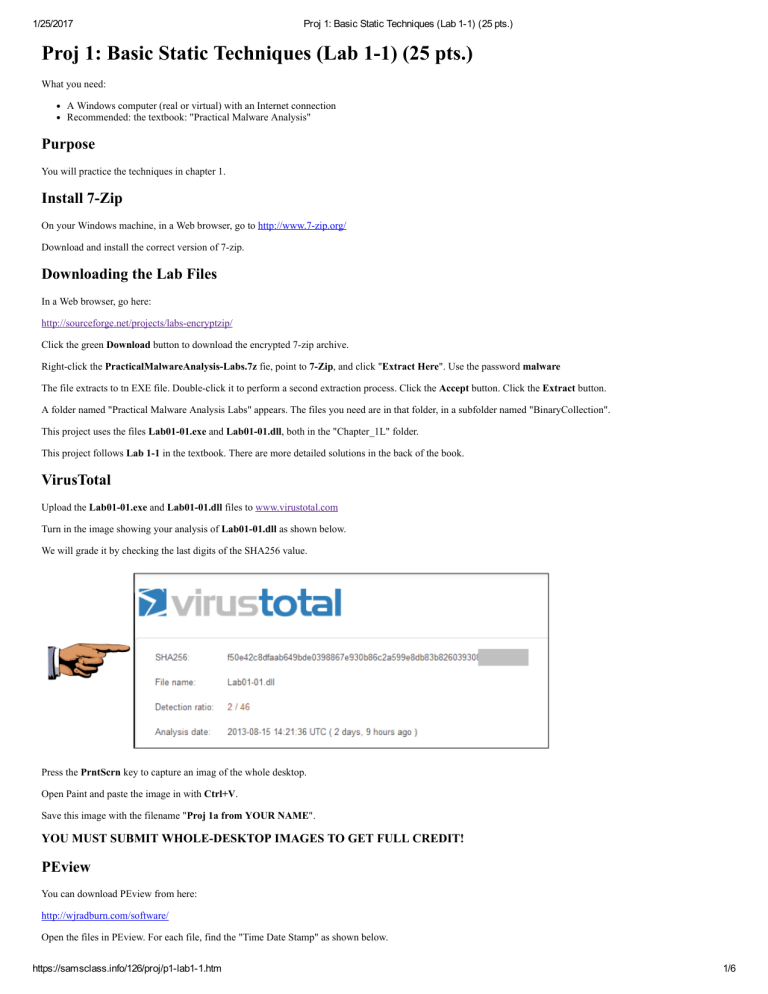This image is a slightly blurred, low-resolution vertical screenshot of a web page with a stark white background. In the top left corner, the date "1/25/2017" is displayed. On the top right, the header reads, "Project 1: Basic Static Techniques Lab 1-1, 25 Points."

The main body of the document is a titled instructional guide labeled "Project 1: Basic Static Techniques Lab 1-1, 25 Points." This document outlines the necessary requirements and steps for completing the project. It specifies that you need a Windows computer (real or virtual) with an internet connection and the “Practical Malware Analysis” textbook. The purpose of the project is to practice the techniques detailed in Chapter 1.

The instructions begin with the installation of 7-Zip software:
- Open a web browser and go to "http://www.7-zip.org".
- Download and install the correct version of 7-Zip for your Windows machine.

Next, it guides on downloading the lab files:
- Navigate to "http://sourceforge.net/project/labs-encrypt.zip" using a web browser.
- Click the green download button to obtain the encrypted 7-Zip archive.
- Right-click on the downloaded "practical_malware_analysis_labs.7z" file.
- Point to 7-Zip and select "Extract Here."
- Use the password "malware" for extraction.

Towards the end, the document references a tool named "VirusTotal," contained within a grayish box with details like "SHA-256," "File Name," "Detection Ratio," and "Analysis Date." The box includes a pen pointing towards it, indicating these are significant aspects to note.

This descriptive caption details the contents and directions provided in the screenshot while offering clarity and context for readers.